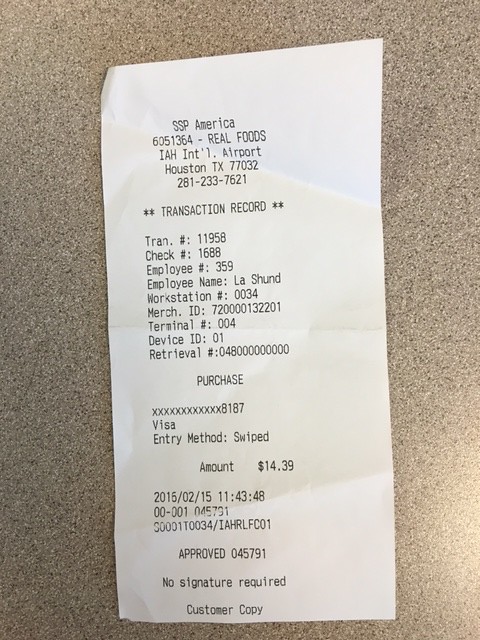This image captures a white, rectangular receipt placed against a grey pebbledash background, likely representing a work surface. At the top of the receipt, the header reads "SSP America" followed by a number and a reference to "Real Foods" at the International Airport Houston. Notably, the receipt does not specify any purchased items, suggesting it might not be a purchase receipt. The inclusion of an entry method, which could indicate a swipe, along with an employee number, implies that the receipt could be related to clocking in, possibly as a record of an employee's sign-in activity.